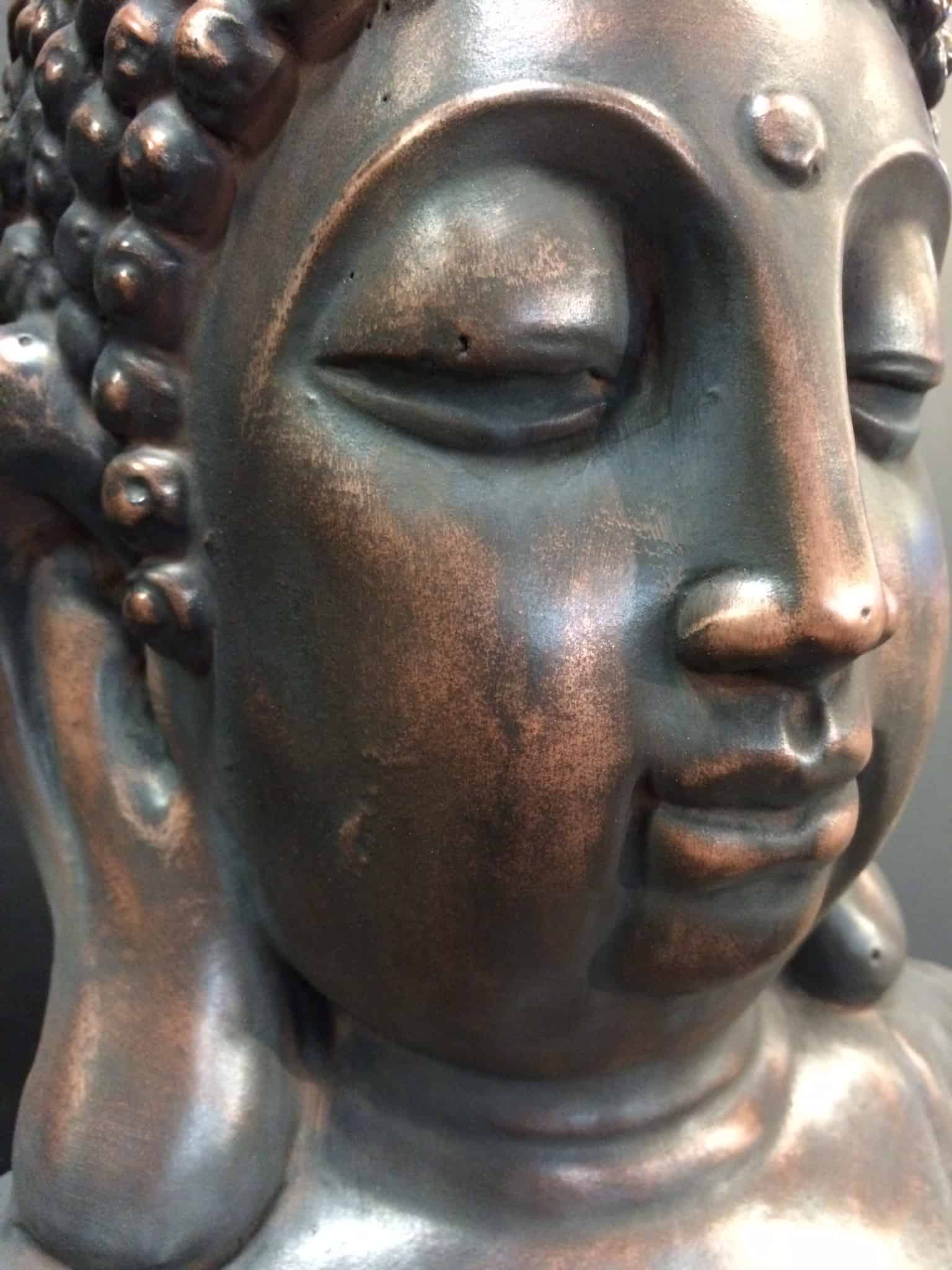This close-up photograph showcases a detailed stone carving of a woman's face, likely representing a figure from ancient times. The face, angled three-quarters to the right, places her right eye, cheek, and mouth in the center of the image, while the left eye and cheek are at the periphery. The stone has a grayish-brown hue with interlaced reddish or rust-colored tones. Her carved features include high-arched brows, heavy eyelids with slightly opened eyes, and rounded cheeks. The nose presents a straight bridge with subtly flared nostrils, and the closed mouth appears relaxed with a faint smile. Intricate beading adorns the area where the hair meets the face on the left side, possibly representing cornrows or braided beads. The hair itself consists of ball-like knobs, indicating tight curls or braids. Large, elongated earrings dangle from the ears, which are sizable and extend down to the neck. The figure's forehead features a distinct, raised circular jewel at the top of the nose bridge. The neck and just a hint of the area below it are visible, merging seamlessly into the rest of the sculpture.